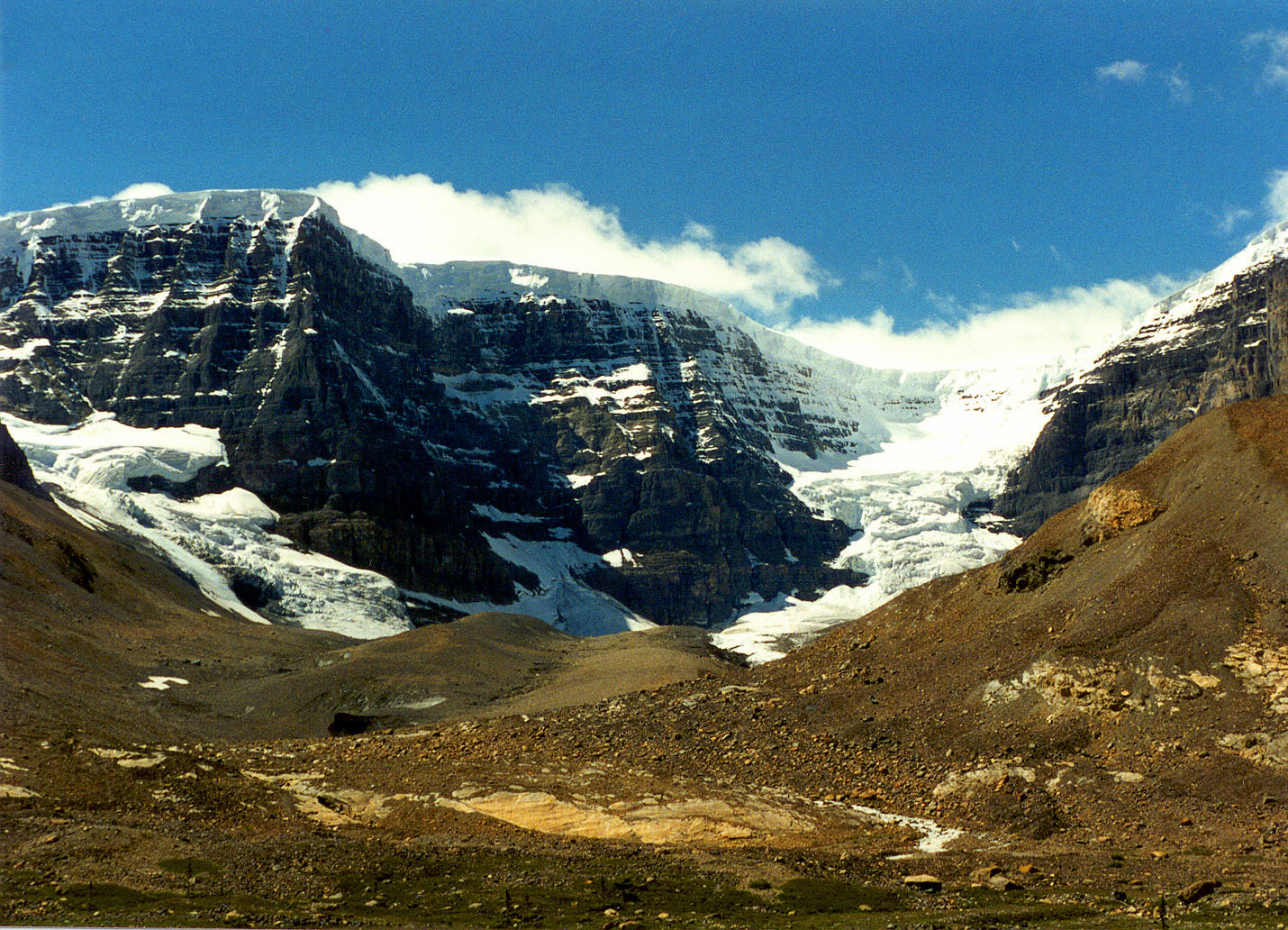This captivating photograph showcases a striking mountainous region, characterized by its high elevation and wintry conditions. The rugged mountain face, composed of stark gray rock, is adorned with snow atop its peaks, with cascades of snow and ice descending the slopes, resembling frozen waterfalls. A prominent glacier adds to the dramatic scenery as it winds its way down the mountain. The lower areas of the image reveal a barren, dirt-filled valley devoid of vegetation, likely cleared by natural forces. The sky above is a mesmerizing expanse of clear blue, dotted with large, billowing cumulus clouds that lazily drift over the majestic landscape. The overall setting is a serene, outdoor daytime scene, enveloped in the splendor of nature’s untouched beauty.